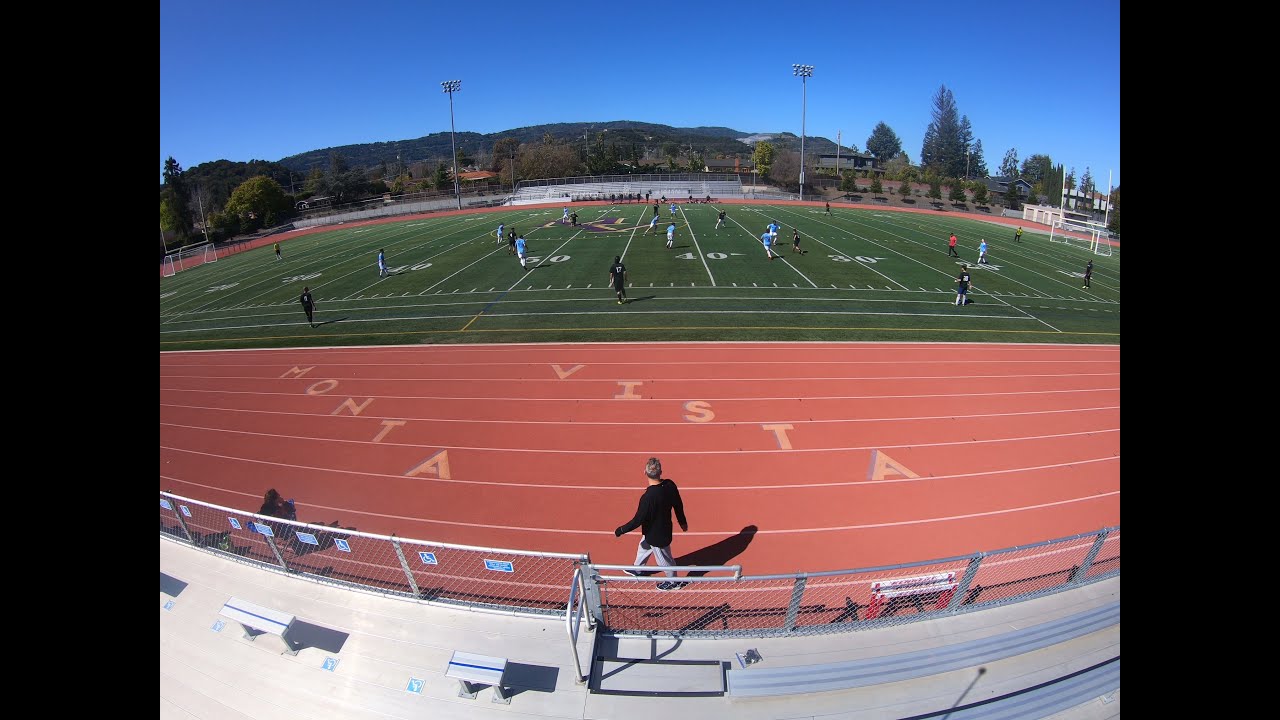This vibrant photograph captures a sunny day at the Monta Vista high school stadium, where athletes can be seen engaging in a lively soccer practice on a green football field. The field is encircled by a striking reddish-brown track, emblazoned with the name "Monta Vista" at a diagonal angle. Two teams are visible on the field: one donning light blue tops with white shorts and white socks, and the other dressed in black tops with matching shorts and socks. A single person in a black sweatshirt walks along the track, gazing toward the ongoing game. Metal bleachers are positioned towards the lower half of the image, hinting at the presence of an audience, while towering stadium lights stand unlit against a remarkably clear, bright blue sky. The backdrop features majestic mountains and an array of evergreen trees, reinforcing the serene beauty of the scene. The angle of the shadows suggests it is midday or early afternoon, bathing the entire stadium in brilliant sunlight.